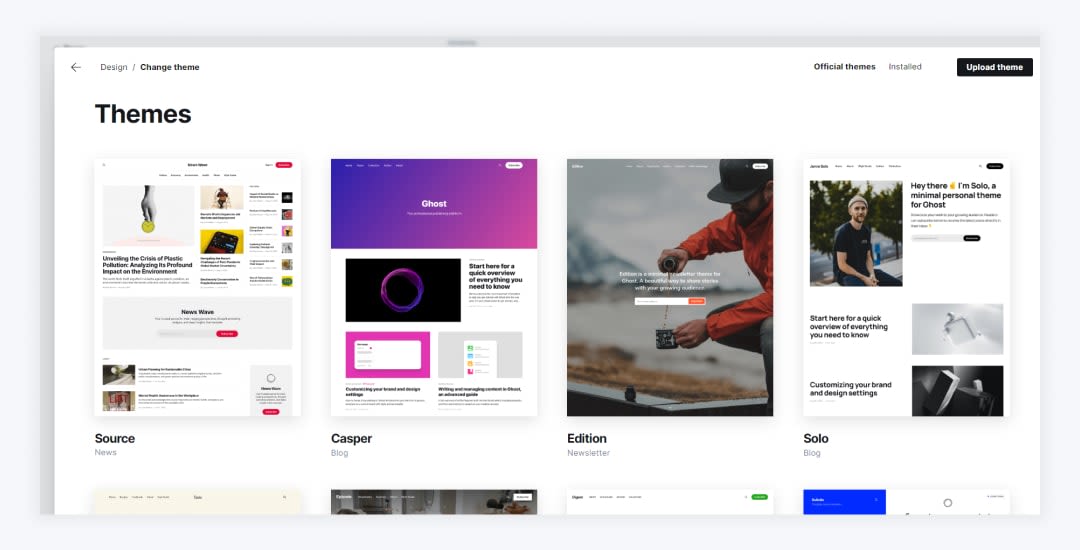In the top left corner of this website, there is a label that reads "Design / Change Themes." On the top right side, there is a section titled "Official Themes" with the options "Installed" and "Upload Theme." The "Upload Theme" option is presented as a black button with white text. The background of the page is white throughout.

Below these sections, there is a larger, bold heading labeled "Themes" in black font. Underneath this heading, there are four rectangular images arranged vertically side by side. Each rectangle features a different theme: "Source News," "Casper Blog," "Edition Newsletter," and "Solo Blog." The text on these images is out of focus and mostly unreadable. 

Beneath the "Solo Blog" theme, there is additional unclear text in blue, seemingly indicating more themes that are partially cut off at the bottom of the screen. The page displays a wide palette of colors including purple, pink, orange, blue, green, white, gray, black, yellow, and red, adding visual variety.

Overall, the page layout focuses on offering various theme options for users, with clear functional sections for theme management and selection.